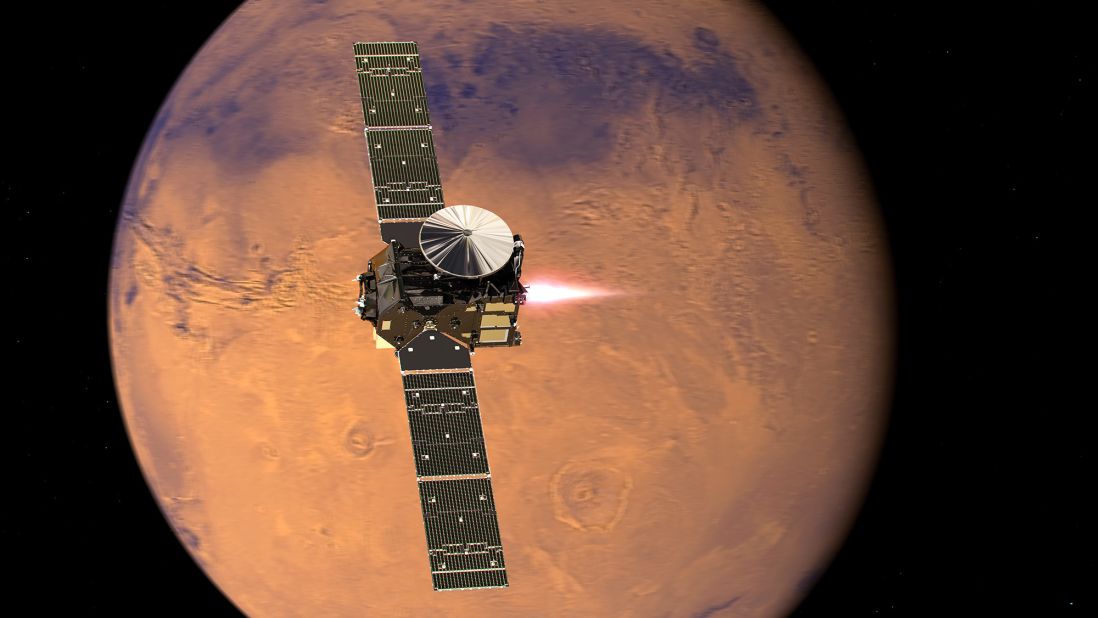The image showcases a satellite orbiting the moon against a stark black background. The satellite, with its metallic silver finish, features a large, shiny, umbrella-like dish antenna at the top, reminiscent of a thumbtack head. Extending from either side of the main squared cube body—adorned with three gold boxes at the back—are long solar panels, two large ones, and a central one shaped like a baseball home plate. The spacecraft is actively firing its rear engine, emitting a pointed flame of orange, yellow, and white. Beneath the satellite, the moon's rugged surface is visible, including a prominent long scar, referred to as the moon's Grand Canyon, surrounded by various craters and a distinct dark area near the top. The moon itself has hues of pink and purplish blue coloring, blending into the cosmic scenery.